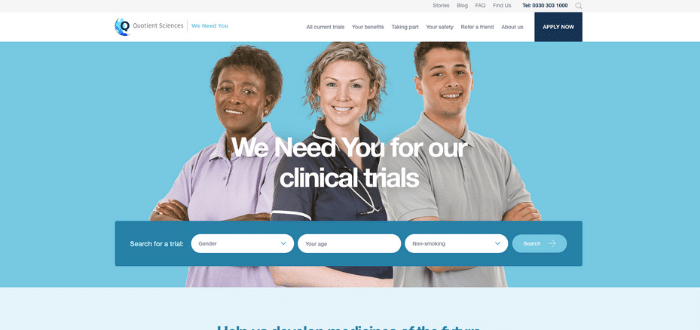Here is a refined and detailed caption for the image:

---

The webpage for Quotient Sciences features a prominently displayed logo at the top left corner, followed by the compelling call to action: "We Need You." The top navigation bar includes options for "Stories," "Blog," "FAQ," "Find Us," and features a telephone number that is currently blurred and illegible. Below this navigation bar are hyperlinks labeled "All Current," "Your Benefits," "Taking Part," "Your Safety," "Refer a Friend," and "About Us." On the upper-right side of the screen, a blue-highlighted "Apply" button in white text stands out.

The main content area of the page features an image depicting three diverse individuals: a black woman, a white woman, and a white man from left to right. Superimposed text reads, "We Need You for our clinical trials." Directly below this, a search box titled "Search for a Trial" allows potential participants to filter clinical trials based on gender, age, smoking status, and other parameters, with an additional search button to refine the results.

---

This caption provides a comprehensive description of the webpage, highlighting key elements and functionalities.